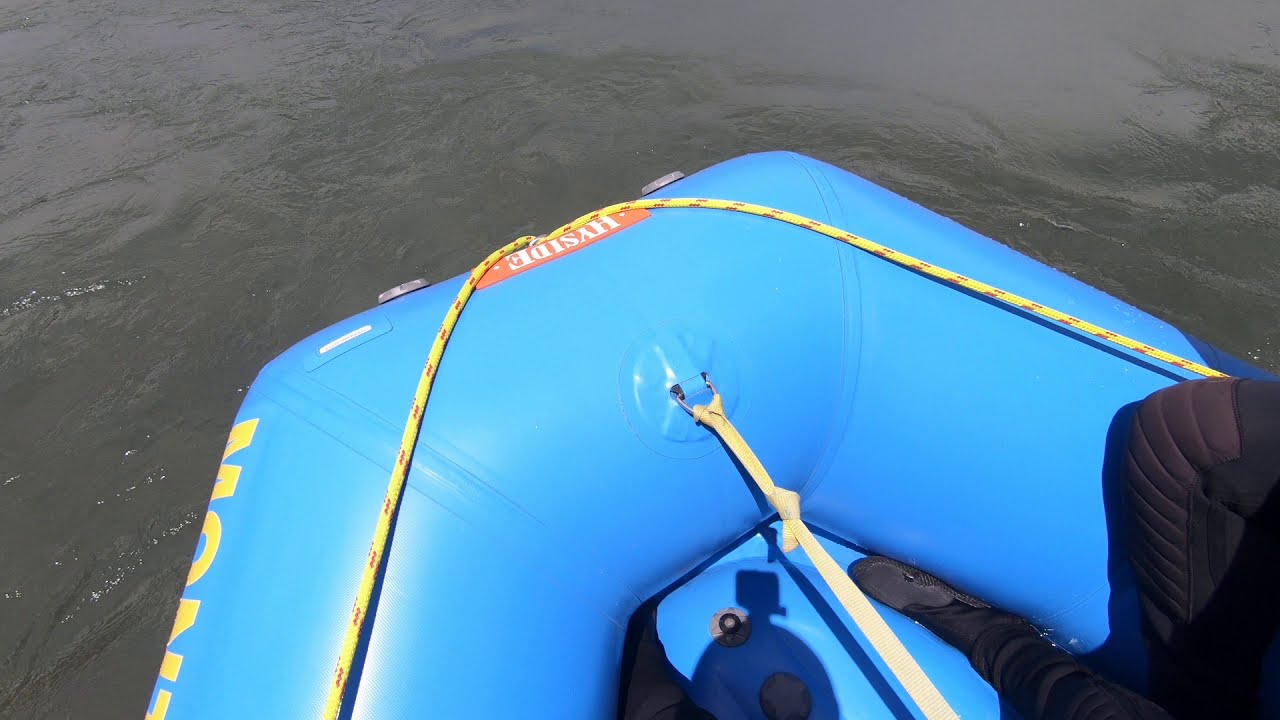The image captures the bow of a bright blue, inflated rubber raft as it gently moves down a calm river. The water, a greenish-gray hue, reflects the sunny sky, suggesting a clear day. The photograph appears to be taken from the perspective of someone sitting at the front of the raft, looking straight down. Prominently featured is a yellow rope with red specks running through it, looped and tethered to both sides of the nose of the boat. In the very center of the bow, a yellow strap is attached to a metal ring. There are two reflectors at the forefront, and an orange badge with the white text "HYSIDE" is slightly visible. The boat has partial yellow writing on the side, which reads "M-O-N-T," but the full name is obscured. The lower right corner of the image reveals a hint of a person’s leg or knee, partially covered in dark clothing with visible padding.